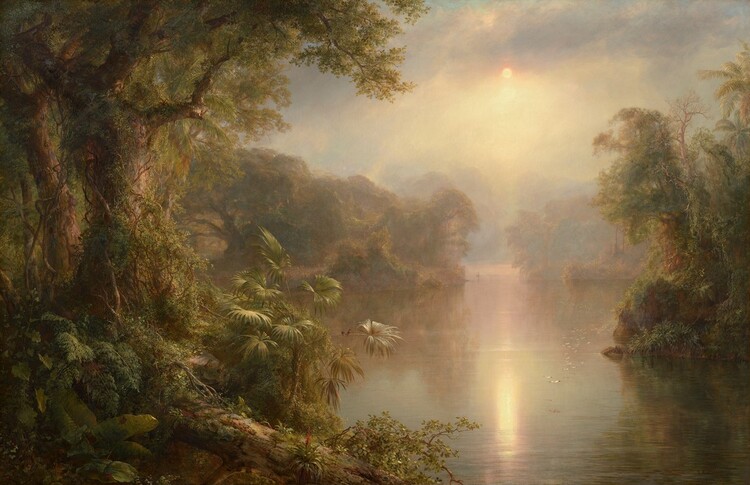This image captures a serene, swamp-like lake at the break of dawn, bathed in muted, natural tones that evoke a quiet, almost mystical atmosphere. A light fog drifts lazily above the still, brown water, rendering the scene misty and atmospheric. The sun peeks timidly through a thick cover of clouds, casting a gentle reflection on the lake's placid surface and subtly illuminating the surrounding landscape.

The edges of the lake are densely populated with trees, many of which are draped in Spanish moss, adding to the swampy, overgrown aesthetic. Moss climbs up their trunks, enhancing the sense of untamed wilderness. There is a palpable stillness in the image; no animals, people, or boats disturb the tranquility. The sky overhead is equally somber, with a heavy cloud cover that mutes the light, reinforcing the early morning, foggy ambiance.

The scene could easily be mistaken for a fine painting, perhaps reminiscent of a southern United States swamp, like those found in Louisiana, complete with diverse vegetation and an air of untouched beauty.